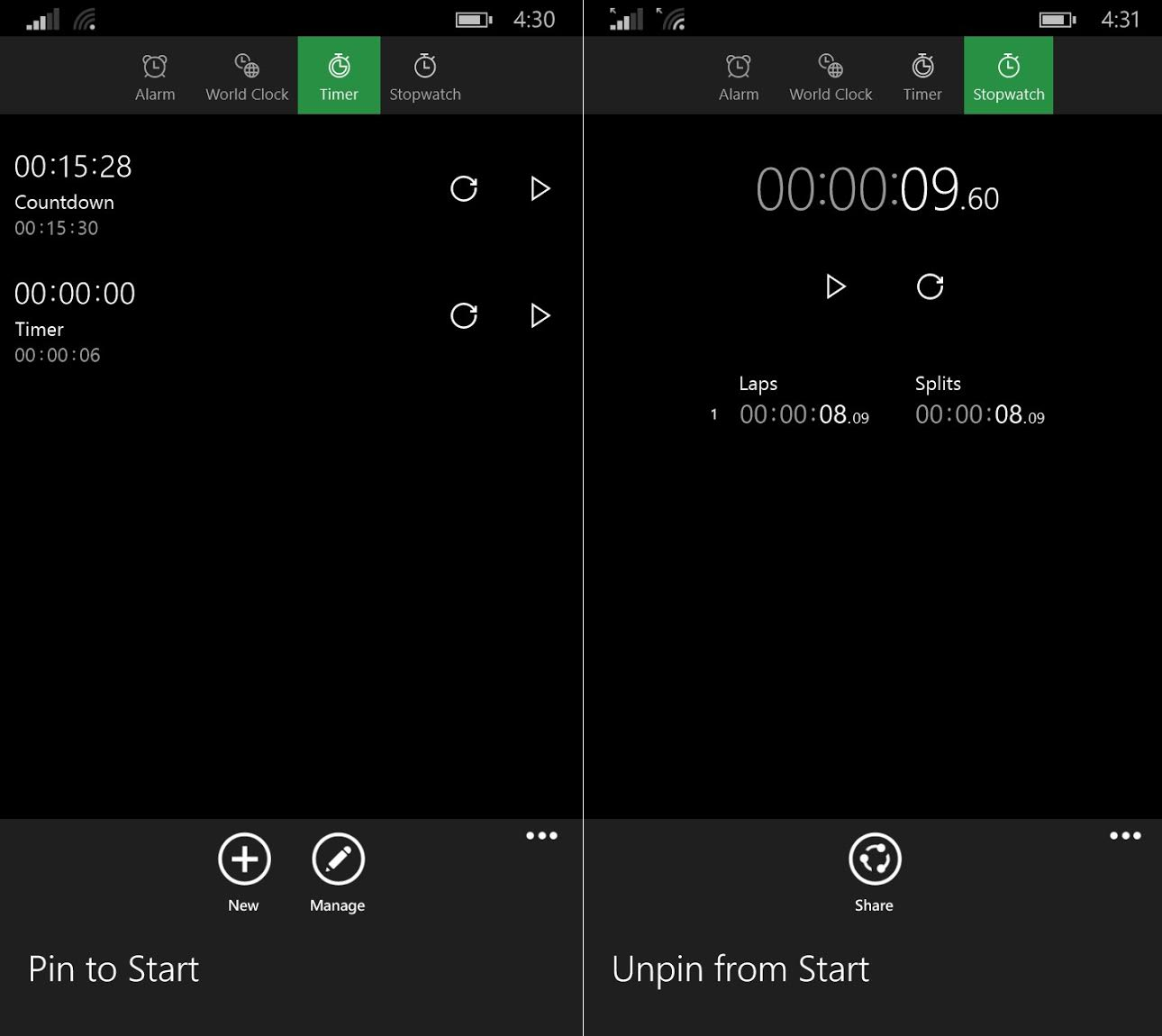This caption accompanies an image featuring two side-by-side screenshots of an iPhone's alarm panel in dark mode. The left screenshot showcases the Timer section. At the top, it displays "15 minutes" beside the label "Countdown," accompanied by refresh and play icons. Below this, the timer shows "00:00:00," with a smaller grey print stating "6 seconds" underneath. To the right of "6 seconds" are refresh and arrow buttons. At the bottom of this panel, a plus icon accompanies the label "New," while a pencil icon next to "Manage" and a "Pin to Start" button are found at the bottom right.

In contrast, the right screenshot highlights the Stopwatch feature. It displays a running time of "9.60 seconds" at the top. Underneath, plus and refresh icons serve to start and reset the stopwatch, respectively. The section below shows "Lapse 8.09" on the left and "Splits 08.09" on the right. At the bottom center is a "Share" icon, with "Unpin from Start" located at the bottom left.